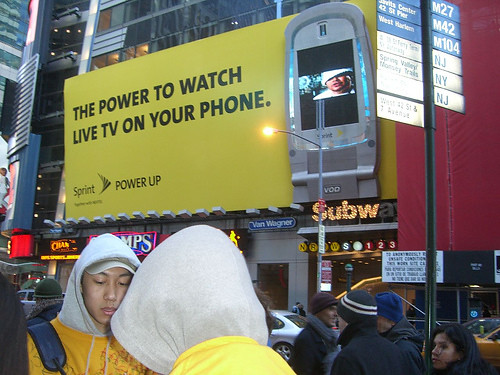In this color photograph, a bustling New York City street scene is captured in vivid detail. Dominating the background, a large, yellow Sprint billboard hangs against the backdrop of towering high-rise buildings. The billboard message reads, "The power to watch live TV on your phone," with the tagline “Sprint Power Up” beneath it, and features an image of a silver flip phone with its screen lit up. Below the advertisement, several shop signs are visible, including a partially illuminated Subway sign and a Champs Sports sign, which is lit up in white with a red border.

Amidst the urban hustle, numerous pedestrians move along the busy street. Notably, two young men stand near a shop, both dressed in light gray hoodies with yellow t-shirts over them—one of them carrying a backpack. They appear to be wearing baseball caps under their hoods, with one of the men possibly of Asian descent. In the background, a yellow taxi cab weaves through traffic, and a notable street sign displays information for routes M27, M42, M104, NJ, and NY, likely indicating nearby transit options. The street is lively with people dressed in winter attire—black coats and knit caps—as they walk past stores and mingle in the vibrant downtown area, highlighting the usual bustle of New York City life.